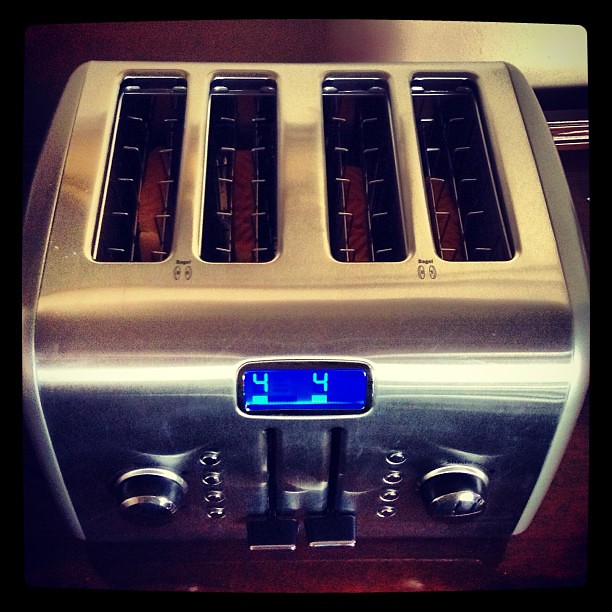This photograph showcases a sleek, stainless steel four-slice toaster with a range of advanced features. The toaster has a gleaming aluminum finish and is positioned prominently in a kitchen setting on a wooden counter. The image, taken from a slight angle above, shows the toaster in operation with four pieces of bread being toasted.

On top, there are four toasting slots arranged widthwise rather than lengthwise, each currently filled with bread. The front of the toaster features a small digital display with two lighter blue '4s' on a dark blue background, indicating the toasting progress. Below the display are multiple controls: two larger knobs with black stripes for adjusting toast darkness, two spring-loaded levers for lowering the bread into the heating mechanism, and eight smaller buttons spaced equally on either side of the knobs. These buttons are used for various functions, likely including settings for different types of bread and other toasting preferences.

The toaster also includes sliding levers in the center that move up and down, possibly for additional control over the toasting process. The stainless steel material adds a modern touch, and the apparatus is designed with user-friendly features for precision toasting. The background includes a tan-colored wall that seems to partially fall into shadow, adding depth to the scene without detracting from the focus on the toaster.